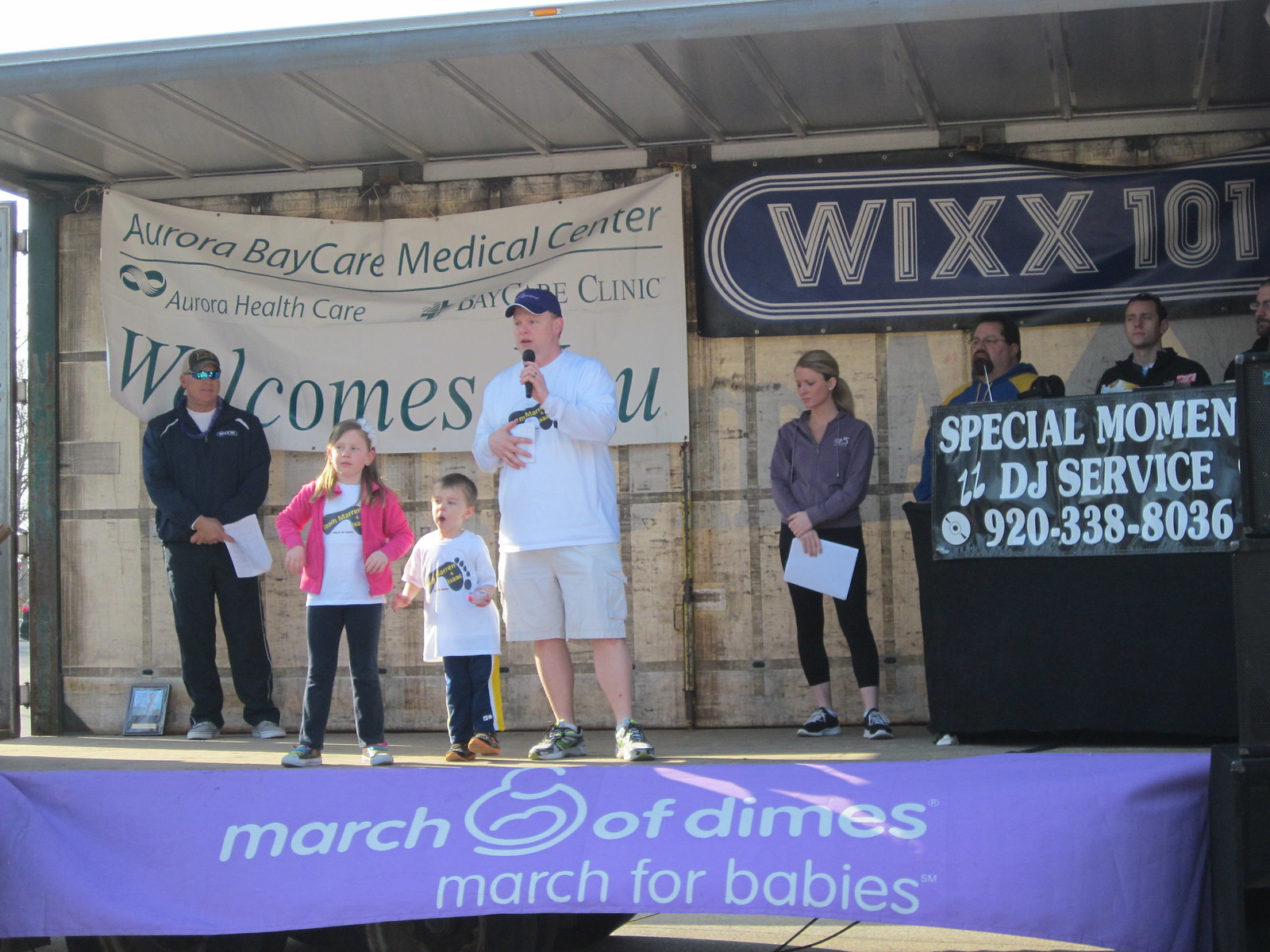The photograph is taken outside at a small stage event dedicated to the March of Dimes March for Babies. The stage has a covered roof and several banners and signs displayed in the background and foreground. At the center of the stage, a gentleman dressed in a white t-shirt and white shorts is holding a microphone. Two kids, a little boy and a girl, stand to his left. 

To the left of the main group, another gentleman in a blue uniform wearing a sun visor is holding a piece of paper. Positioned behind him is a large banner that reads “Aurora Bay Care Medical Center welcomes you” in white and green font. On the right side of the stage, a woman holding a piece of paper stands under a black sign that features "WIXX101" in a blue oval with white font.

At the front edge of the stage, there's a large purple banner with light blue writing stating "March of Dimes, March for Babies." Additionally, a small table on stage bears a sign for "Special Women DJ Service" with the phone number 920-338-8036. Three people are standing behind this table. The overall scene captures a moment from an outdoor charity event, showing a diverse group of participants and a well-branded stage setup.